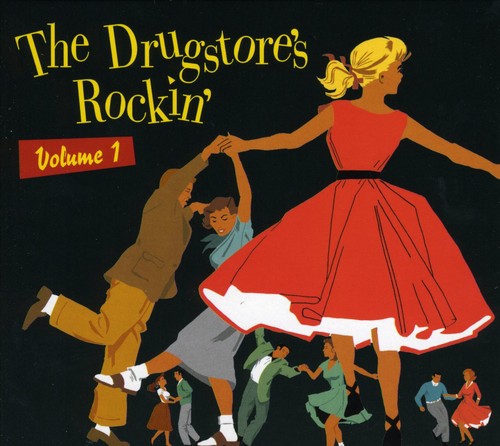The album cover image for "The Drugstore Rockin' Volume 1" features a vibrant illustration with a black background. Yellow text at the top left reads "THE DRUGSTORE'S ROCKIN'", with the letters slightly uneven, followed by a red banner that contains the text "VOLUME 1" in yellow. The focal point is a cartoon depiction of a blonde girl in a strapless red dress and black belt that poofs out to her knees, with black shoes and a white lining inside the dress's bottom. She is prominently dancing in the foreground, holding hands with two other characters: a man dressed in a brown jacket, brown pants, brown shoes, and white socks, and a woman in a blue shirt, gray skirt, brown sandals, and white socks. Surrounding them are graphical images of couples dancing in 1950s and 1960s attire, including men in suits and women in long dresses with fitted tops. The overall color palette includes greens, reds, and browns, contributing to a lively depiction of mid-20th-century dance culture.